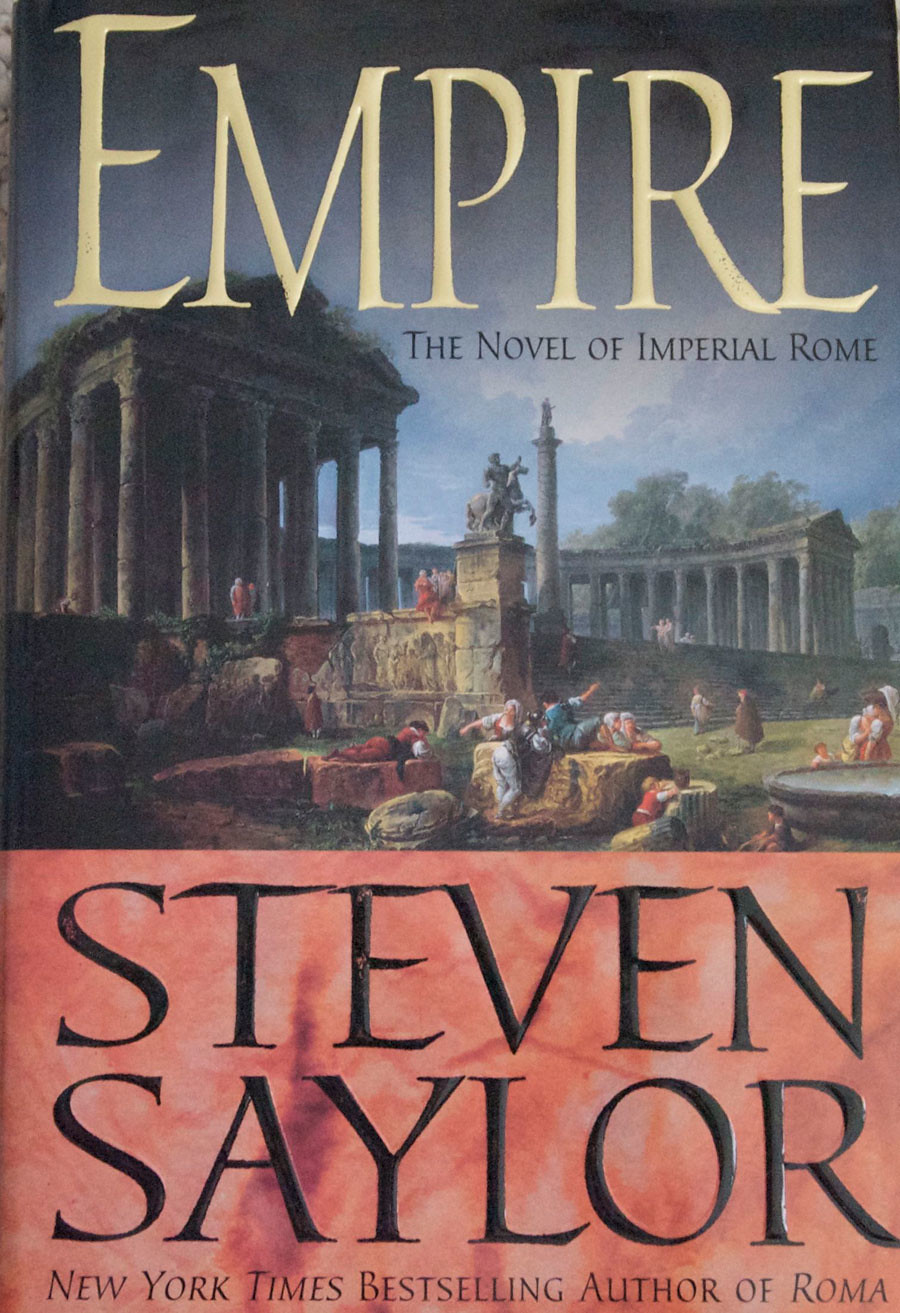The image is a detailed scan of a fictional paperback book cover. The top half of the cover features an elaborate painting depicting Roman ruins with various people engaging in recreational activities. The scene showcases a U-shaped building abundant with large marble columns, steps, and structures with triangular roofs. Statues on pillars, a fountain, and numerous individuals in robes epitomize the iconic imagery of ancient Rome. In raised gold lettering at the very top, the title reads "Empire, the novel of Imperial Rome." The bottom half of the cover is adorned with a pinkish banner mimicking stone texture with dark pink splotches. Prominently displayed in semi-raised black text are the words "Stephen Saylor, New York Times bestselling author of Roma."